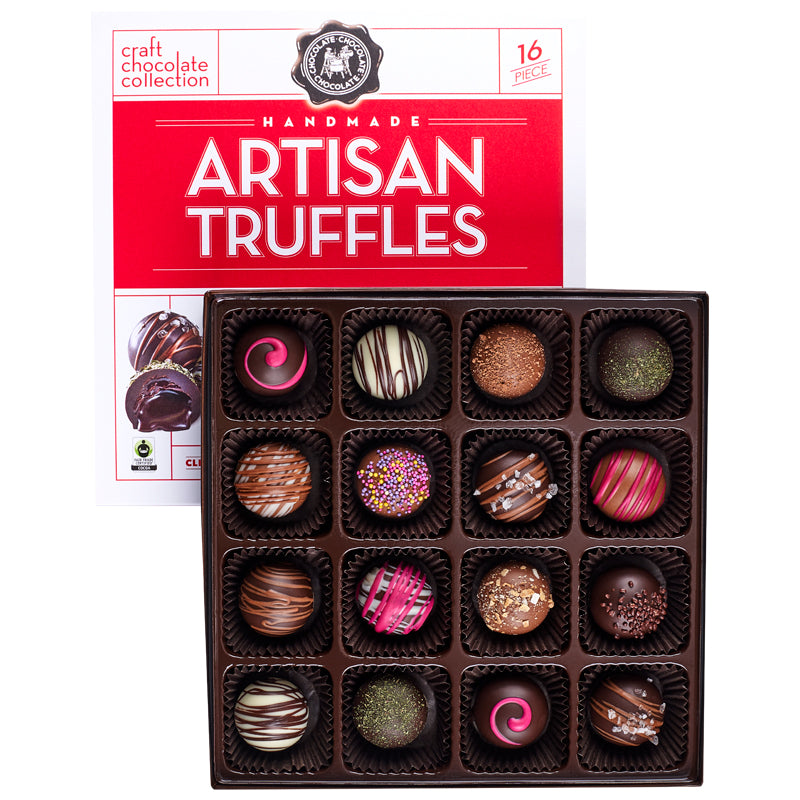This image showcases an open box of handmade artisan truffles, neatly arranged in four rows of four, totaling 16 pieces. The assortment includes various colors and designs, featuring brown chocolates with pink swirls, white chocolates with dark stripes, and an array of other truffles in pink, green, white, gray, and brown. The chocolates come with diverse toppings, like sprinkles, swirls, and salted caramel. 

The box's cover, which is partially visible underneath the open container, has distinct red and white elements. In the top left corner, it features a red outline and the text "Kraft Chocolate Collection" in red. In the center of the cover, a black circle with a white interior displays the brand's emblem. The top right corner prominently states "16 piece" in red text. Below, a red banner with white lettering declares them "Handmade," followed by a larger text proclaiming "Artisan Truffles." The cover also displays images of two truffles in the lower portion, mostly obscured by the dark brown container holding the chocolates. This promotional image emphasizes the variety and artisanal quality of the truffles.